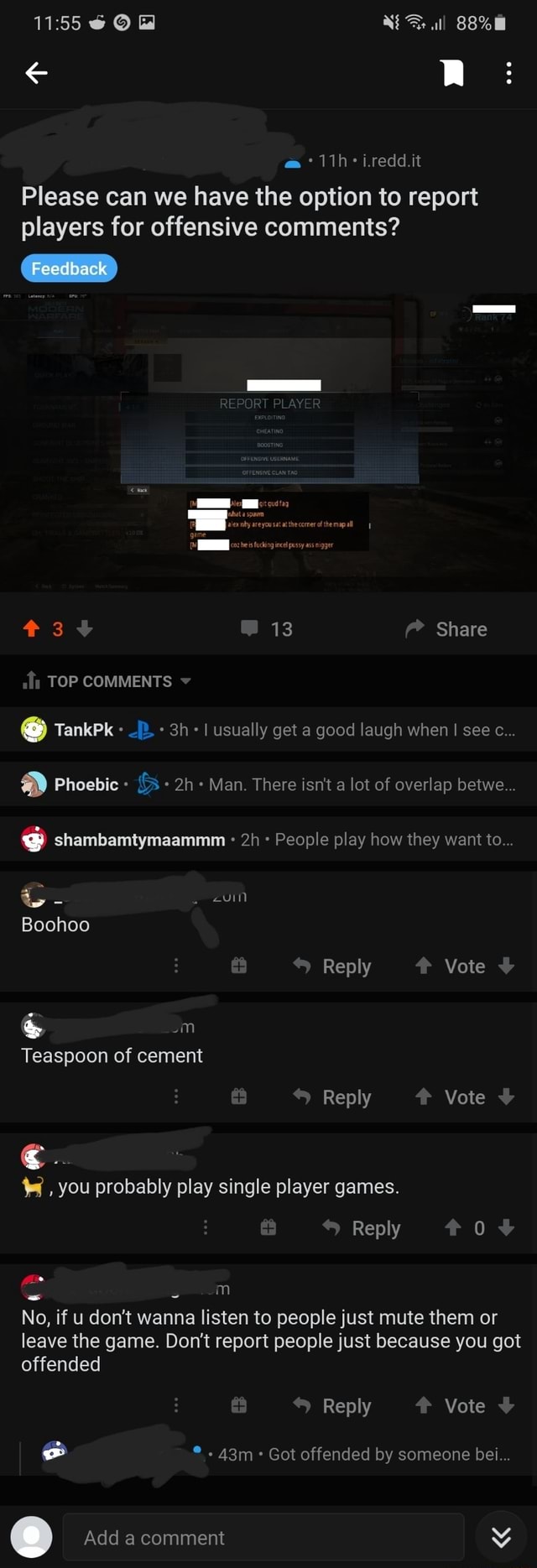The image is a clear screenshot taken from a cell phone. At the top of the image, the status bar displays the time as 11:55, accompanied by three icons. On the right side of the status bar, there is a Wi-Fi icon, a few other indistinguishable icons, and a battery icon displaying an 88% charge.

Just below the status bar, on the far right, there's a bookmark icon, though it's unclear if it's activated or not. On the left side, there's a left-pointing arrow for navigation.

The main content of the screenshot shows a conversation or feedback section. At the top, there's a text stating, "Please can we have the option to report players for offensive comments," accompanied by a blue tag labeled "feedback." 

Below this text, several comments are displayed, though most are not easily readable. The image indicates that there are six different responses, some of which include images that are not clearly visible.

At the very bottom of the screen, there's a bar for user interaction that says "Add a comment."